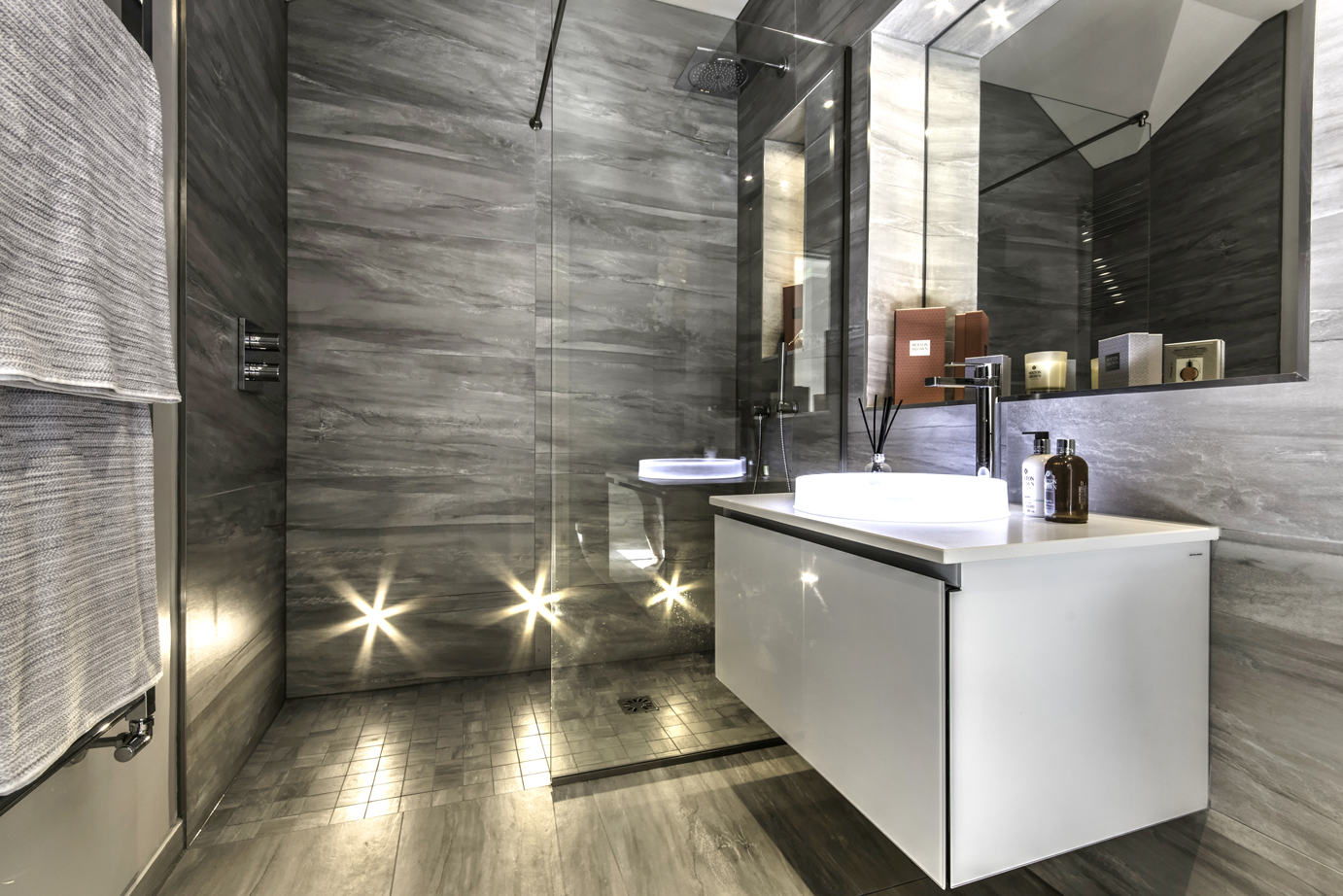This image showcases a luxurious and modern bathroom predominantly featuring shades of gray and white. The centerpiece is a spacious shower adorned with marble-like tiles incorporating hints of purple. A trio of yellow star-shaped lights illuminates the base of the shower, enhancing the elegant ambiance. The shower is enclosed with a high, transparent glass panel that extends from the floor to ceiling, separating it from the adjacent white-cabinet-mounted sink. The sink area, topped with a white counter, holds several brown and white bottles. Above the sink, a well-arranged mirror reflects multiple items, including boxes and a candle. On the left side of the image, the wall incorporates both the shower knobs and horizontally patterned gray and white curtains. The bathroom floor features gray and white wood-grained tiles, adding to the overall sophisticated aesthetic, hinting that this space belongs to someone of considerable wealth.